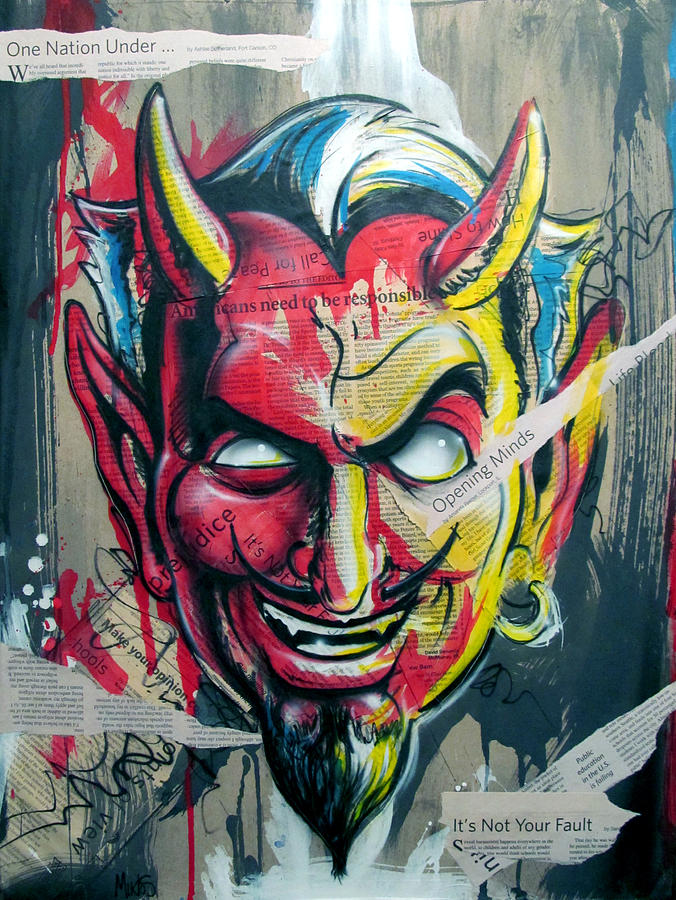The image is a vertical, rectangular art collage featuring a prominent, creepy depiction of a devil in the center. The devil mask is primarily red with yellow accents and has distinct, white, empty eyes. It has blue and white hair, a pointed mustache shaped almost like an exaggerated smiley face, a goatee, and pointy teeth. The horns of the devil are red, yellow, and black. The background consists of smeared paint strokes in black, gray, beige, and red, adding to the eerie atmosphere.

Interspersed throughout the collage are several ripped newspaper clippings. Notable texts include "One Nation Under" at the top, "Opening Minds" next to one of the eyes, and "It's Not Your Fault" in the bottom right-hand corner. Additionally, there are clippings with smaller text that are difficult to read. This multi-layered composition, with its unsettling central figure and chaotic background elements, evokes a sense of discomfort and introspection.